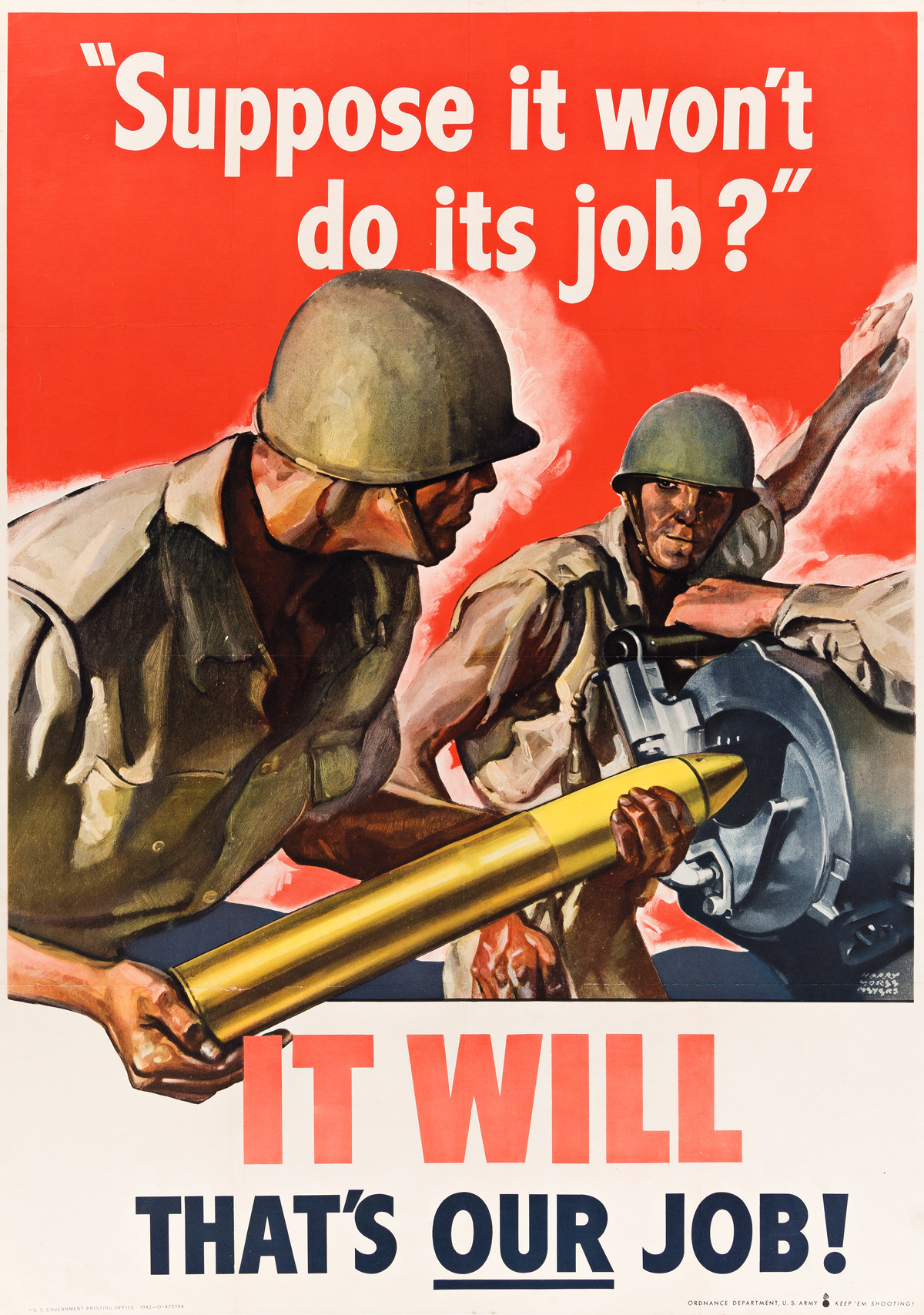This World War II era military propaganda poster features a vivid red background with bold white lettering at the top, reading "Suppose it won't do its job." The central illustration is a detailed painting of two soldiers in green military uniforms and helmets. One soldier, closer to the front, is seen from the side holding a large, gold-colored missile, preparing to load it into an artillery gun held by an unseen third person whose arm is just visible. The second soldier is watching the first as he performs this task. Both soldiers' appearances include distinct details like visible skin and one with dirt on his face, adding to the realism of the scene. Below the illustration, on a white background with red and blue text, it declares, "It will. That's our job!", with "our" notably underlined for emphasis. White clouds or smoke add depth and context to the setting, enhancing the poster's gripping and motivational message.